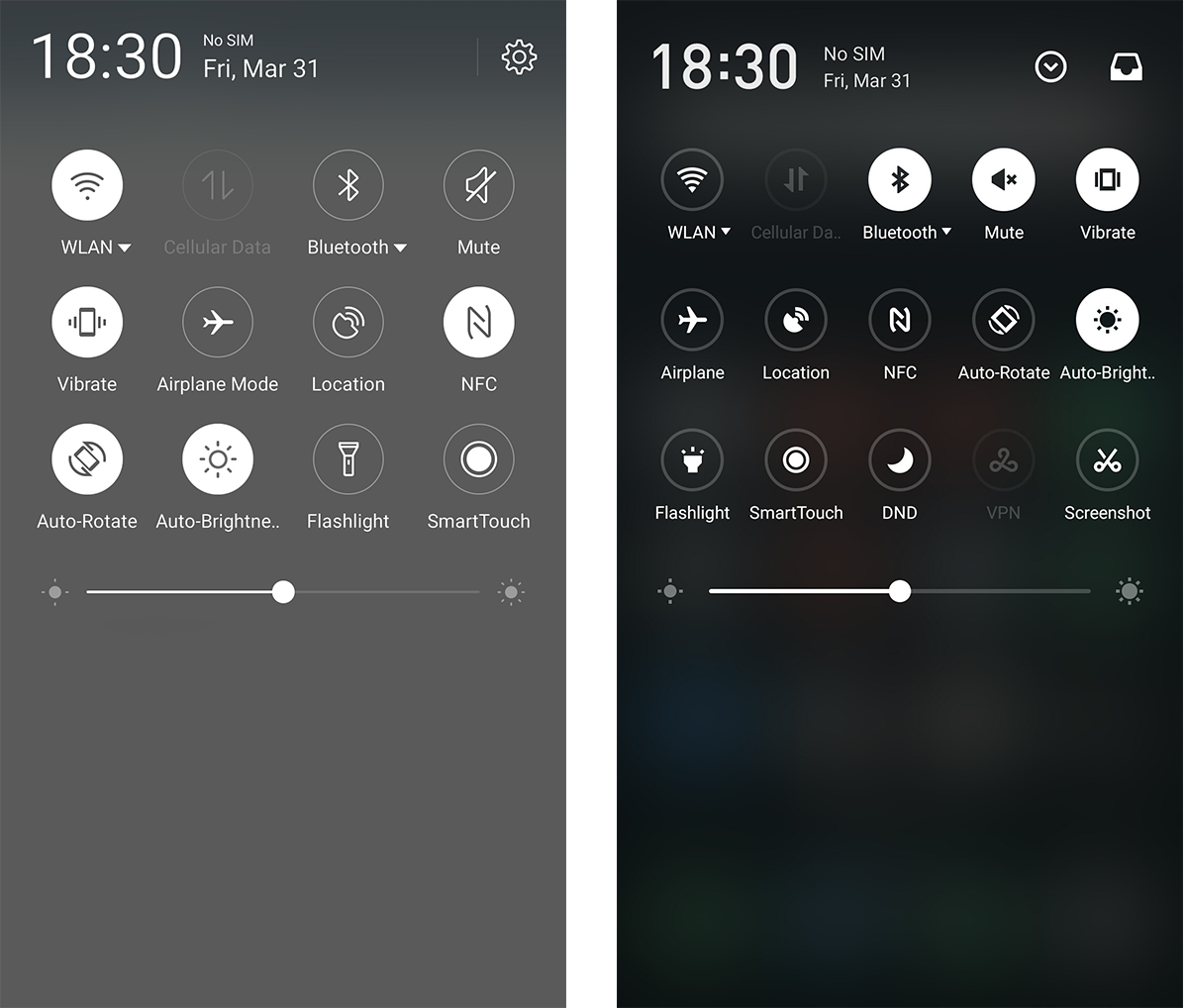A screenshot displaying a mobile phone's quick settings menu with a predominantly gray and black background. The time "18:30" is prominently shown, along with the date "Friday, March 31." The status bar indicates "No SIM" and active connectivity options such as "WLAN," which is highlighted in white, while other icons like cellular data, Bluetooth, mute, vibrate, airplane mode, location, NFC, auto-rotate, auto-brightness, flashlight, and smart touch are mostly in gray. The brightness slider is positioned midway.

The second screenshot, also with a black background and the same date and time, shows slight variations. The "WLAN" icon is now gray, while Bluetooth, mute, vibrate, and the auto-brightness feature (abbreviated as "VRIGHT...") are switched to white, indicating they are active. Both screenshots display the same system control icons, depicting a comprehensive view of the phone's current settings in various modes.